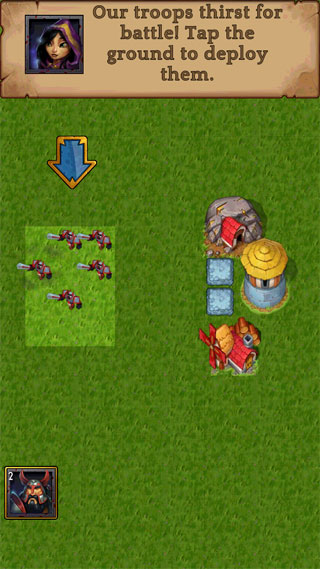This image is a screen capture from a mobile game in a small rectangle format designed for smartphones. The top portion of the image features a beige bar with a weathered paper texture. In the top-left corner of this bar is a small avatar of a pale woman with black hair, depicted from the shoulders up. She wears a purple and yellow wizard's hood. The bar also contains brown text that states, "Our troops thirst for battle! Tap the ground to deploy them."

Below this section, the background transitions to a verdant expanse of variegated green cartoon grass, occupying approximately three-fourths of the image. A blue arrow with yellow edging points towards a group of six small figures wielding knives or swords. These figures, depicted in shades of red and gray, stand ready for deployment.

To the right of these troops, several structures are depicted against the green field. These include two huts, one with a red roof and one with a yellow roof, as well as a barn with a windmill. Additionally, there are two white square blocks and two blue square blocks, possibly representing unidentified elements of the game’s environment. In the bottom-left corner, a box contains an image of a man wearing a helmet, adding further to the game's detailed interface.